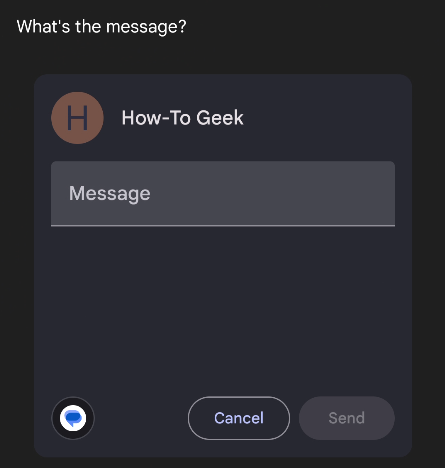The image captures a user interface for a messaging application on a device. The background of the interface is predominantly black, featuring a large square with a solid black background in the top left corner, displaying the text "What's the message?" in white lettering, followed by a question mark.

Below this, there is a slightly lighter black or dark gray background square. At its top, the username "HowToGeek" is displayed. To the left of the username, there is a brown circular icon with an uppercase black "H" in the center, representing the user’s profile image or icon.

Underneath the username, there is a message input box in light gray, with the placeholder text "Message" in white lettering. No message has been typed in this box.

In the lower left corner of the screenshot, the Google Messages icon is visible, characterized by a white circle with a blue word bubble inside. To the right of this icon are two buttons: "Cancel" on the left and "Send" on the right. The "Send" button, along with its lettering, appears grayed out, indicating it is currently inactive and unclickable since no message has been entered in the text area.

Overall, the image provides a detailed snapshot of a minimalist, dark-themed messaging interface in a paused state, awaiting user interaction.